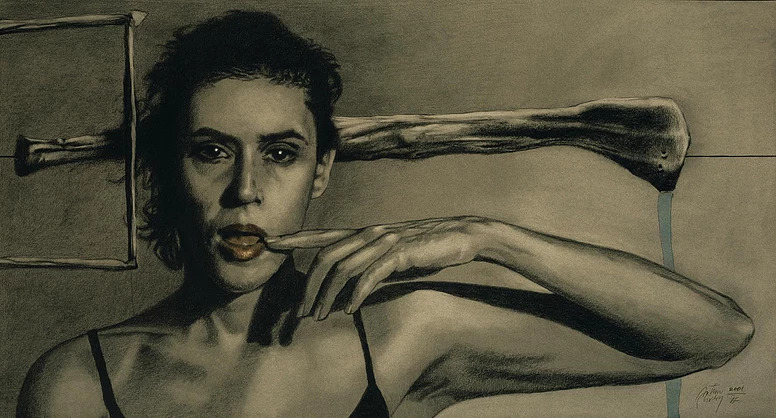The artwork is a horizontal image reminiscent of a film screen, featuring a central figure that is likely a woman, characterized by her distinctive red lipstick. This striking red against the black and white and shades of gray composition makes the lips particularly noticeable. The woman, with very deep black eyes highlighted by a white shine in the middle, and dark black hair, is positioned centrally within the piece. She holds her left arm up and bent at the elbow, with her finger teasingly pointing towards her open mouth, revealing her tongue. Surrounding her are various objects, including a large bone motif that horizontally spans the background, and what appears to be an empty frame to the left. A light blue stripe runs down from the bone to the bottom of the image, adding a subtle color accent. At the bottom right, the artist's signature is visible, yet there is no other text present. The overall style suggests a painting, possibly watercolor or oil-based, rich in suggestive imagery, and the composition implies a refined, gallery-worthy aesthetic.